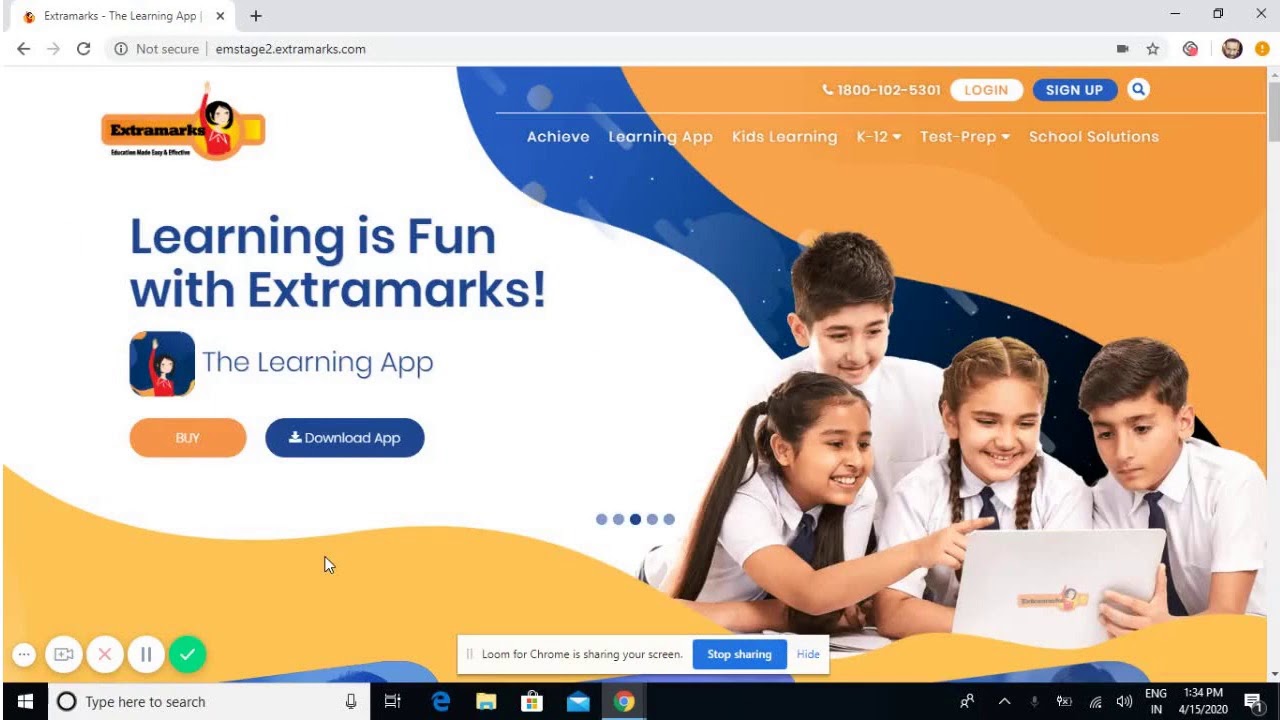This screenshot captures the homepage of the ExtraMarkz website, a dedicated learning app. In the top left corner, the logo reads "ExtraMarkz: The Learning App," with the web address entered in the address bar beneath it. At the center of the page, a prominent image features four children, all attired in short-sleeved white shirts, gathered closely around a laptop. On the left, a girl with pigtails is seen pointing at the screen and smiling, with a boy standing behind her also smiling as he looks at the screen. Directly in front of the laptop, another girl with pigtails, dressed in a white shirt and black tie, focuses intently on the screen. To her right, a boy is equally engaged with the content on the laptop, though his expression is neutral.

On the far right side of the image, there is a text overlay that reads "Learning is fun with ExtraMarkz." Adjacent to this text is an icon of a square featuring a child in a red shirt raising their hand against a blue background. Beneath the icon, there are two prominent buttons: an orange "Buy" button and a blue "Download App" button.

In the upper right section of the page, additional text informs users about the app's offerings, which include "Achieve Learning App, Kids Learning K through 12, Test Prep, and School Solutions." Above this description, a contact phone number is listed, followed by "Login" and "Sign Up" buttons, suggesting easy access to the platform's user interface.